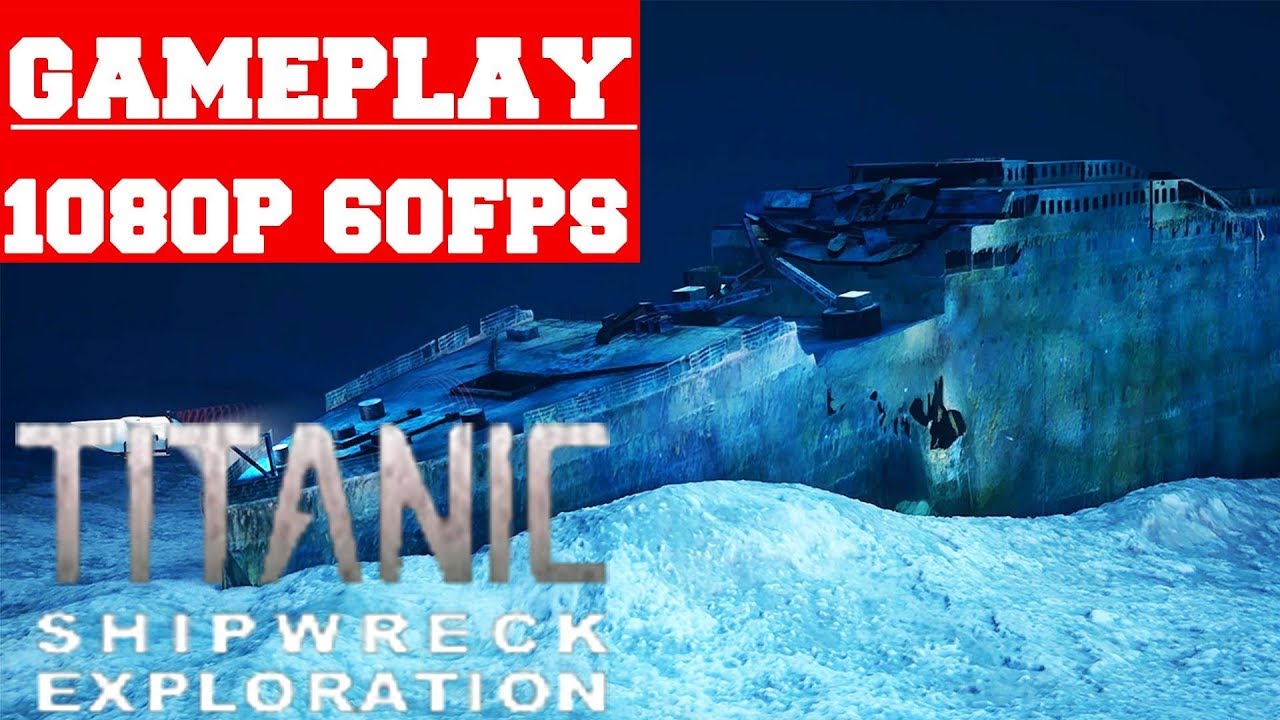The image depicts a gameplay simulation of the legendary Titanic resting on the ocean floor. The ocean in the background is almost black, creating an eerie and spooky ambiance. The Titanic is rendered in shades of blue and dark blue, with slight accents of white, highlighting its ghostly presence underwater. Sand can be seen in the foreground, possibly accumulated over years against the ship’s hull. 

In the top left corner of the image, bold white uppercase text on a striking red background reads "Gameplay." Below it, in the same white text, it says "1080P 60FPS," indicating the resolution and frame rate of the simulation. Directly over the bow of the ship, written in gray uppercase letters, is the word "TITANIC." Beneath this, in white capital letters, it says "SHIPWRECK EXPLORATION," reinforcing the theme of the game. The bow of the Titanic is positioned on the left, with the rest of the wreckage trailing to the right, emphasizing the fragmentation of the vessel. The primary colors in the image are deep blues, complemented by touches of red and white from the text, offering a clear yet somber depiction of the sunken ship.